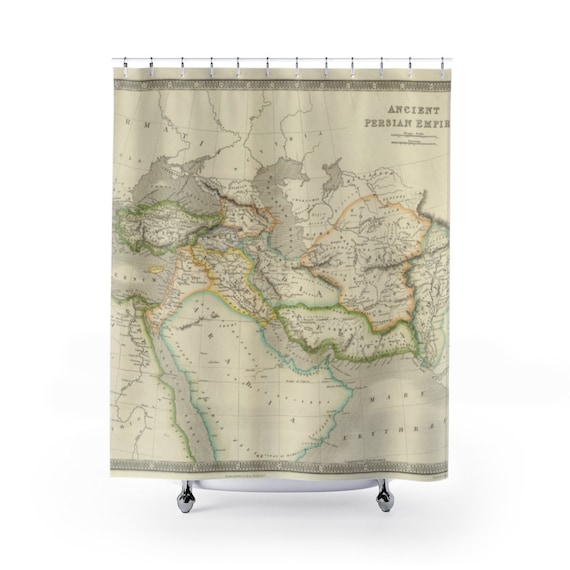This image features a detailed product photo of a beige-colored shower curtain displaying a historical map of the ancient Persian Empire. The curtain, secured by small metal hangers on a rod, covers a white bathtub with visible metal legs. The map on the curtain is predominantly gray with outlined regions in green, red, orange, and yellow, with landmasses highlighted in tan and red, and water bodies shown in gray. Various areas of the map are labeled with text, although the writing is not easily readable. The top right corner of the map prominently displays the dark brown text "Ancient Persian Empire." The overall scene contrasts the white background and bathtub with the intricate, multicolored historical map design of the shower curtain.